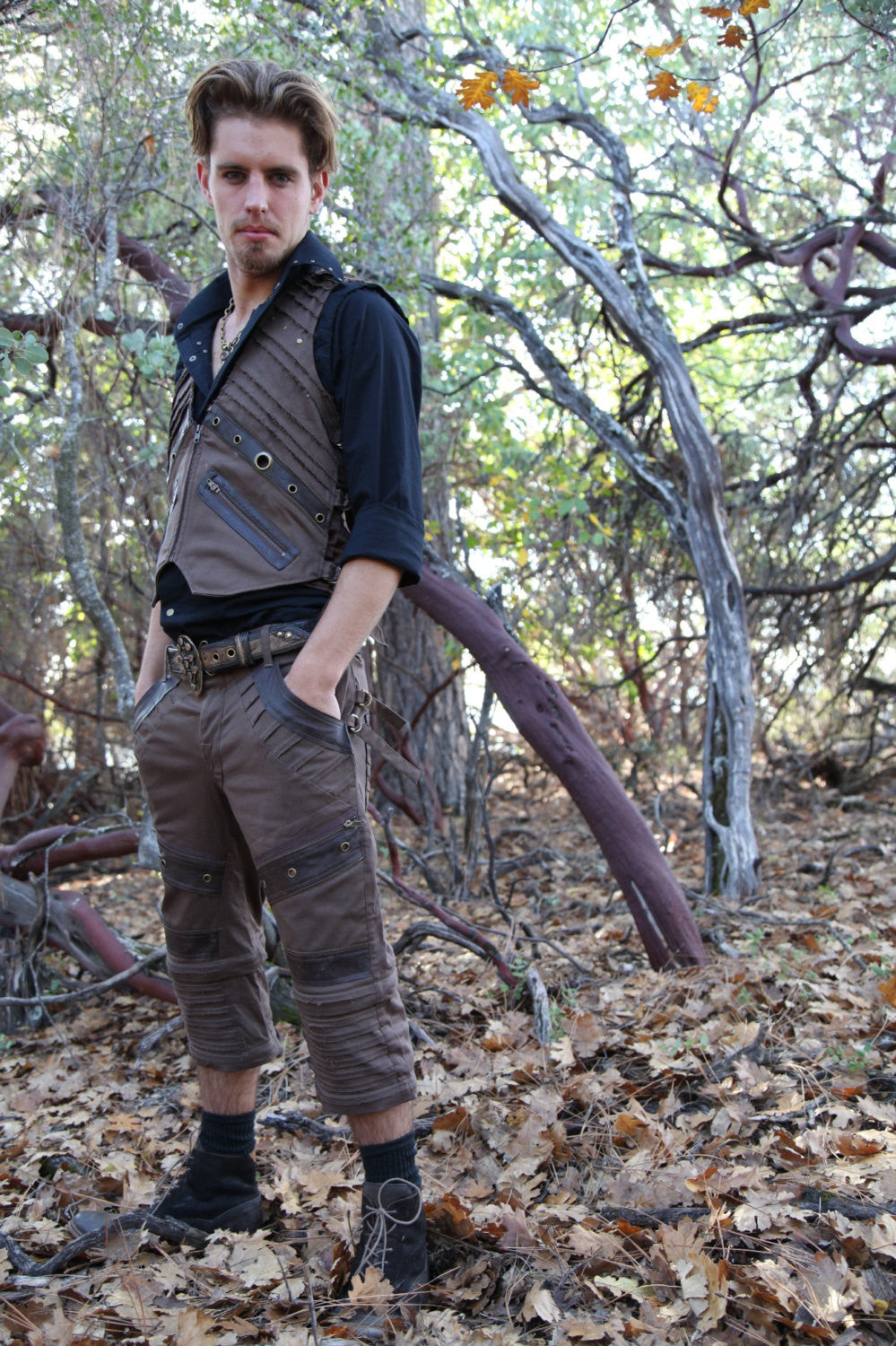The image captures a male model standing in a dense wooded area with twisted, curly branches and a forest floor covered in brown leaves, suggesting an autumn setting. The model has poofy, short brown hair and a brown goatee, and he stands upright with a serious expression, looking directly at the camera. He wears a steampunk-inspired ensemble, consisting of short, brown pants that end at the shins with rivets and cross bracing fabric, paired with black socks and black boots. His outfit also includes a black shirt with rolled-up sleeves and a matching brown vest and belt. The light filters through the trees, illuminating the scene with a foreboding yet intriguing ambiance.